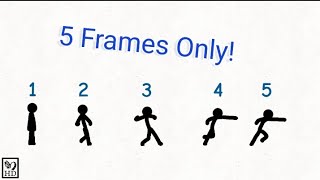The image is a landscape-oriented diagram set against a predominantly white background, with a thin black border running along the top. Below this border, the phrase "five frames only!" is prominently displayed in blue, albeit slightly angled. The diagram is arranged horizontally and comprises five sequentially numbered frames, each featuring a black stick figure illustration. 

- In frame 1, labeled with a blue number "1," the stick figure stands upright.
- Frame 2, marked with a blue "2," shows the figure with arms out to the sides and one leg lifted.
- In frame 3, denoted by a blue "3," the stick figure has its arms spread out and legs apart.
- Frame 4, bearing a blue "4," depicts the figure with one arm and leg extended forward, suggesting a throwing motion.
- Frame 5, indicated by a blue "5," shows the figure stepping forward, completing the throwing action.

This sequence seems to illustrate a simple animation or instructional guide on how to bowl. Additionally, the bottom left corner of the image contains a small "HD" logo inside a square.